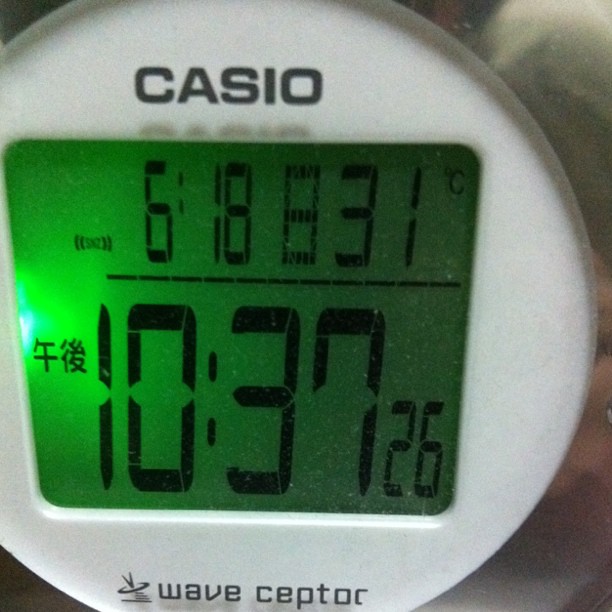This image features a white circular digital clock with a green LCD display. The top of the clock face prominently displays the brand name "CASIO" in bold black letters. Below this, the display area is divided into several sections: in the upper part is a green square with a slightly brighter green section on the left center, showing "6:18". Adjacent to this is "31 C", indicating the temperature. The main, primary display at the center reads "10:37:26" in black digits. Below this central time display, to the left side, are two pieces of Chinese calligraphy. At the bottom of the digital display area, the brand name "Wave Scepter" is visible in smaller text. The green hue of the LCD might appear more vivid, possibly due to lighting in the photo.